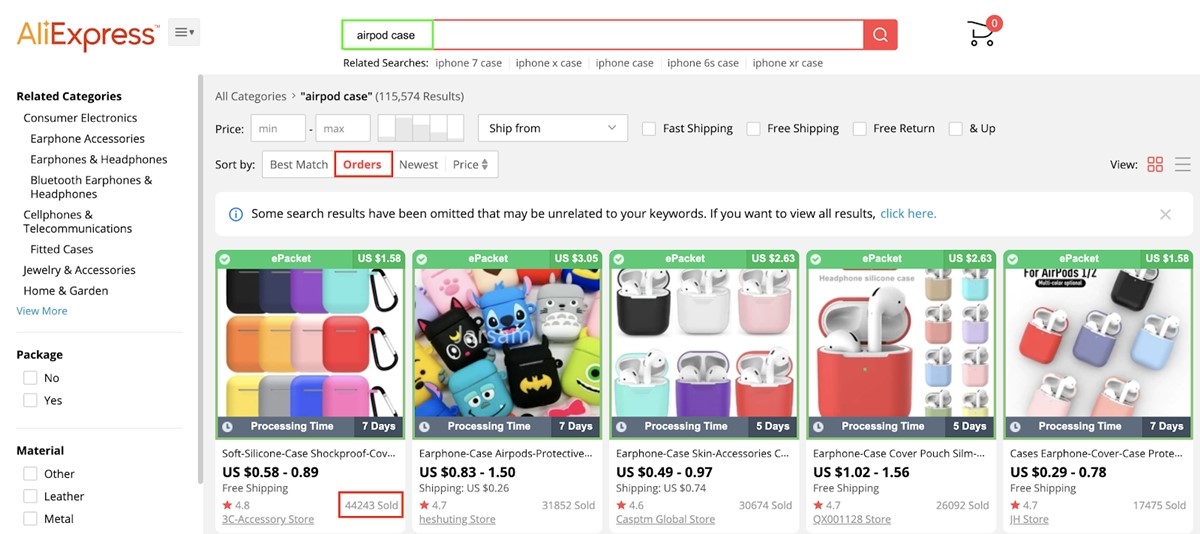A screen capture of an AliExpress webpage showcasing a variety of AirPod cases. The selection includes numerous colorful options, featuring cases equipped with little carabiners for easy attachment to bags or keychains. Among the designs, there are playful ones adorned with different faces, one featuring the Batman symbol, and others available in solid colors including black, white, blue, red, as well as pastel shades like beige and lilac. The display caters to a person looking to purchase a protective and stylish case for their AirPods, turning to AliExpress as their preferred shopping destination.